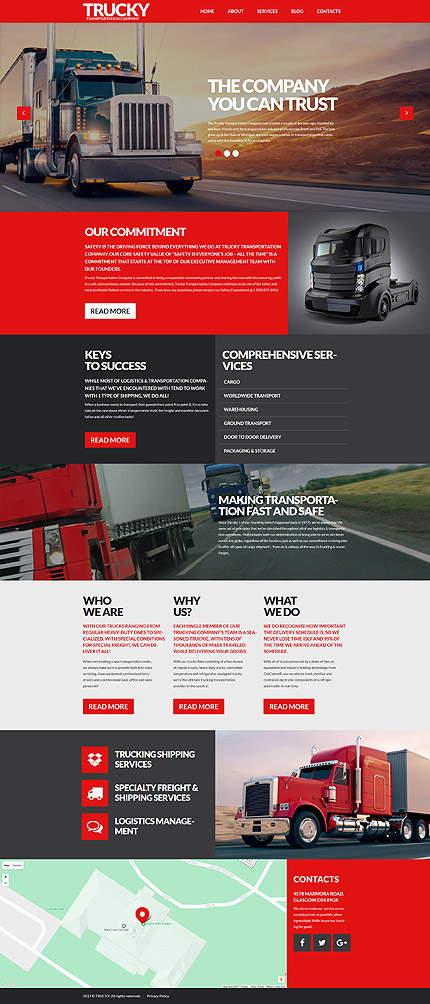The image from the Truckee website features a striking, silver-colored truck cruising down a highway adjacent to a brown hillside. Prominently displayed next to the truck is a red square with the text "Our Commitment." The caption emphasizes the company's trustworthiness, stating, "A Company You Can Trust." Below this, the phrase "Keys to Success and Comprehensive Services" is artfully rendered, with "Keys to Success" in dark gray and "Comprehensive Services" in light gray.

The image transitions into a more extensive visual showing a convoy of trucks: the first truck is red, the second is blue, and the third appears to be gray. Accompanying this visual is the tagline "Making Transportation Fast and Safe." Further down, a white section elucidates the company’s ethos with headings like "Who We Are," "Why Us," and "What Do We Do," each accompanied by detailed explanations.

In a boxed dark gray section to the right, images depict various types of services offered by the company. Adjacent to this is another vivid picture of a real red truck, below which a map is presented, pinpointing a specific building location with the caption "Contact Us."